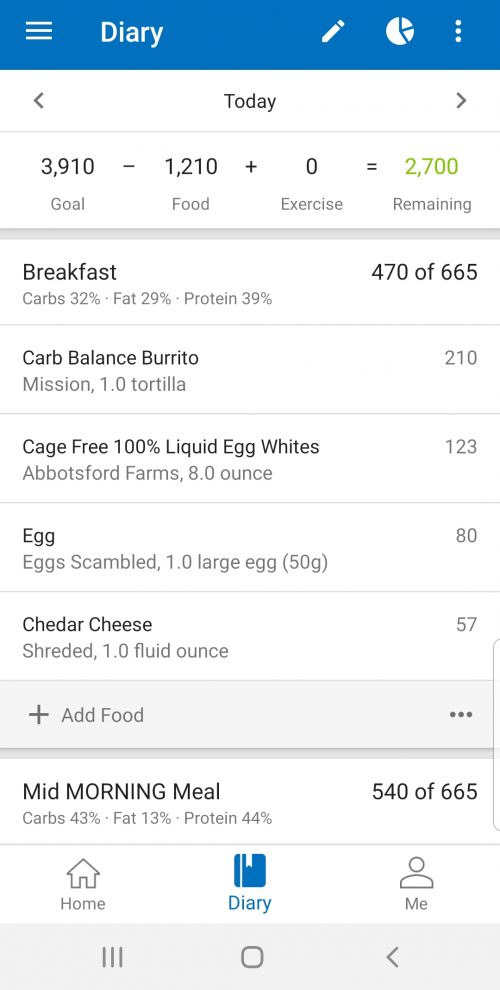This is a detailed screenshot from a diary mobile app. At the top, a blue background bar spans across the image, featuring several functional icons. On the far left is a list button, followed by the word "Diary" centered. To the right, there is a pencil icon for editing and an additional circular icon with three horizontal lines inside, and at the far right, three vertically stacked dots indicating a menu.

Below the blue bar, the background shifts to white. Here, navigation icons include a back button on the left and a forward button on the right, with the word "Today" centered between them. Further down, sections labeled "Goal," "Food," "Exercise," and "Remaining" are visible, outlining various health and fitness data.

The food log includes "Breakfast," listing items such as Carb Balance, eggs, cheese, and their respective calorie counts. At the bottom of the image, there are tabs labeled "Mid-Morning Meal," alongside navigation options "Home," "Diary," and "Me."